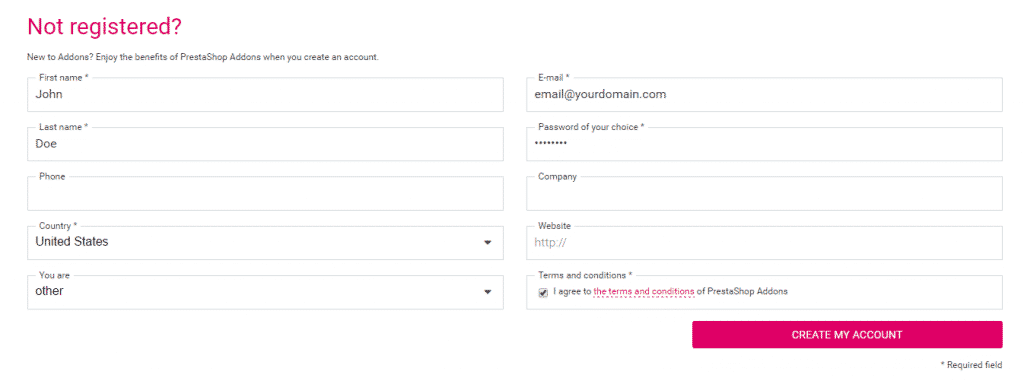This image is a screenshot of a webpage section providing a user registration form on a solid white background with no visible border. At the top left of the form, red text reads "Not registered?" followed by a small black font that appears to say "New to [something]? Enjoy the benefits of [something] Adonis when you create an account." Below this header, the form is divided into two columns containing fields for user information.

The left column includes five input fields with thin gray outlines labeled: 
1. First Name (filled with "John")
2. Last Name (filled with "Doe")
3. Phone
4. Country (set to "United States" with an adjacent dropdown menu for selecting different countries) 
5. You Are (set to "Other" with an adjacent dropdown menu for other options)

The right column comprises additional fields:
1. Email (pre-filled with "email@yourdomain.com")
2. Password (input hidden with asterisks)
3. Company (left blank)
4. Website (partially pre-filled with "http://")
5. Terms and Conditions (a checkbox which is already checked, indicating acceptance)

Certain fields, such as Email, Password, First Name, Last Name, and Country, are marked with asterisks, denoting that they are mandatory for form completion.